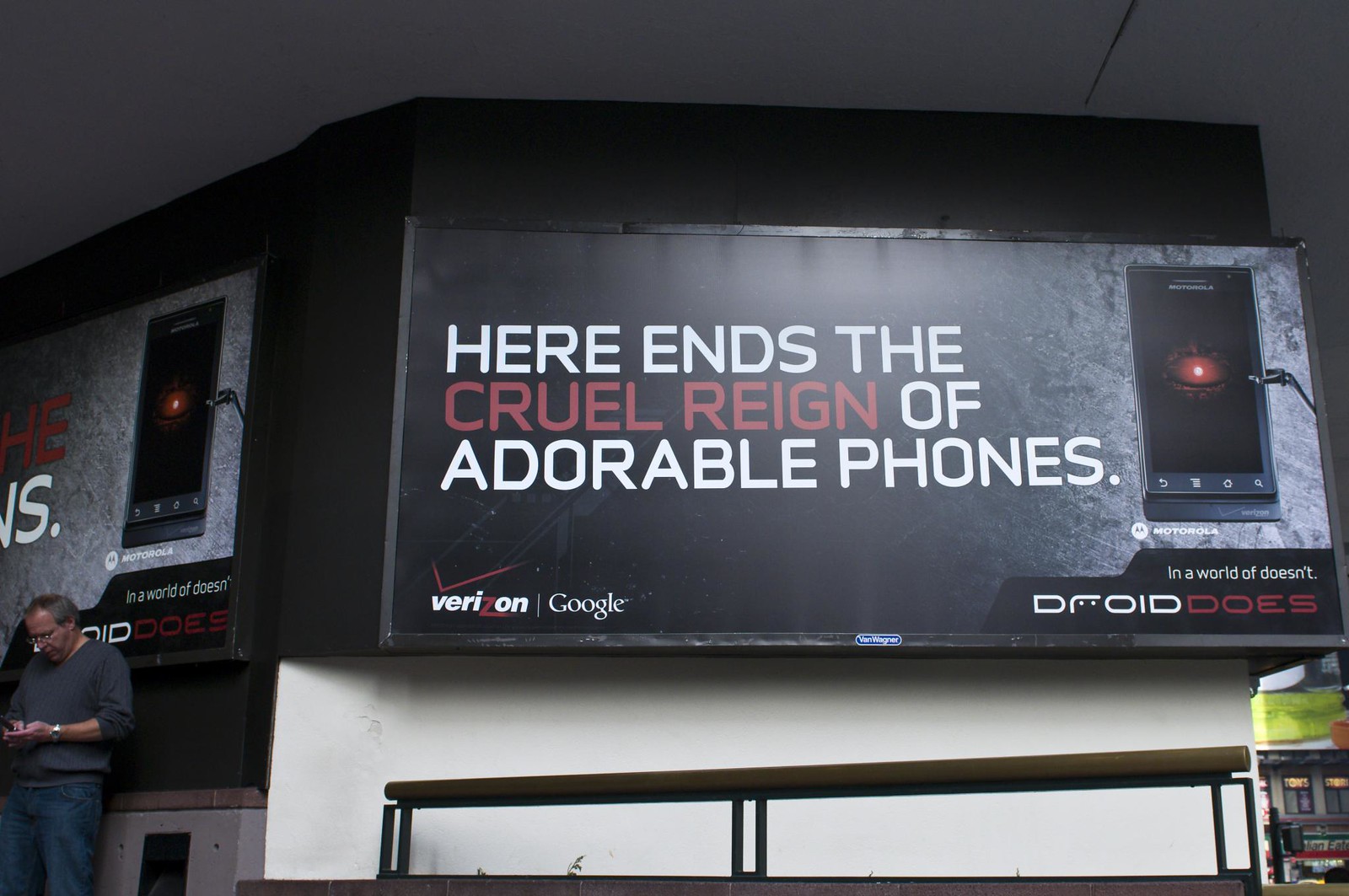In the foreground of the image, a large sign dominates with bold white text on a dark background that declares, "Here ends the cruel reign of adorable phones," with "cruel reign" highlighted in red. The lower left corner of this sign features the Verizon logo and its checkmark, while the word "Google" is displayed to the right. At the bottom right of the sign, the text “Droid” is prominently shown, and beneath that, in red letters, it reads, “In a world of doesn’t, Droid does.” The upper right corner of the sign mimics the screen of a cell phone. 

A man stands towards the lower left side of the image, dressed in a gray, long-sleeved shirt rolled up to his elbows, blue jeans, and what seems to be a silver watch. He is seen looking down at his phone, positioned under the same sign, which curves around to the left side of the picture, providing a different perspective. In front of him, a white barrier runs horizontally, accompanied by a brown wooden board that acts as a divider between his position and the sign. The lower right corner of the picture also includes another depiction of a phone’s screen, adding to the technological theme. Overall, the central theme of the image is the dramatic sign highlighting the end of the "adorable phones" era, emphasizing Verizon and Google's Droid phone.